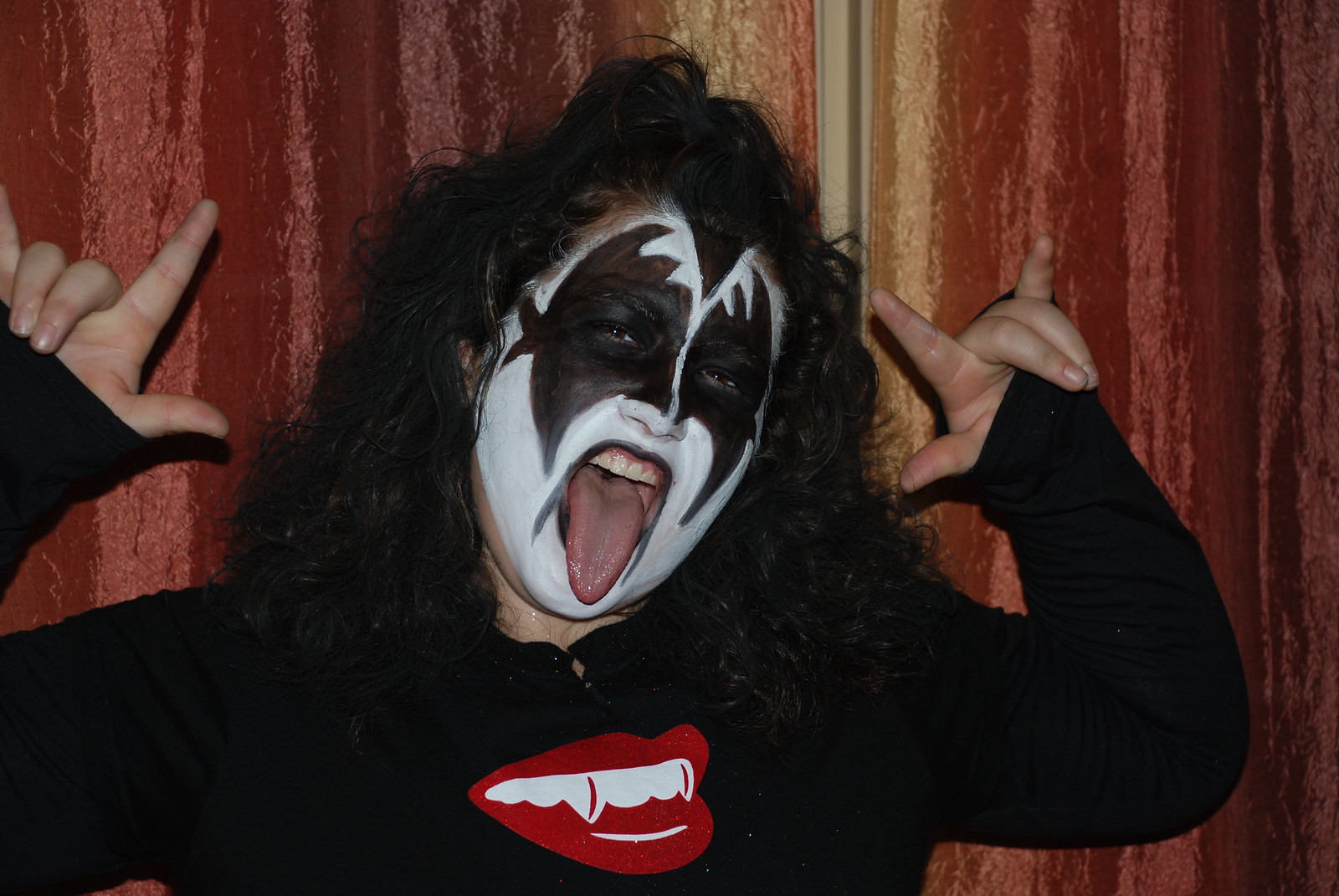A close-up photo captures an individual dressed as Gene Simmons from KISS, standing against a wood-paneled wall with streaks of pink and red in the background. The person, who appears to be light-skinned, has meticulously applied face paint featuring the iconic KISS makeup: a white base with black shapes that extend from the eyes like triangular bat wings, and black-outlined lips that highlight their open mouth and extended tongue, revealing the top row of teeth. The individual sports a black, long-sleeve t-shirt adorned with a graphic of red lips, white teeth, and pronounced fangs accented by red, giving the design a three-dimensional effect. Their black, curly hair is pulled back to frame their face, resembling a wig styled in the fashion of Gene Simmons. Completing the authentic rock 'n' roll look, the person holds their hands on either side of their head, forming the signature devil horns gesture; though the left hand is partly cropped out by the photograph's edge.